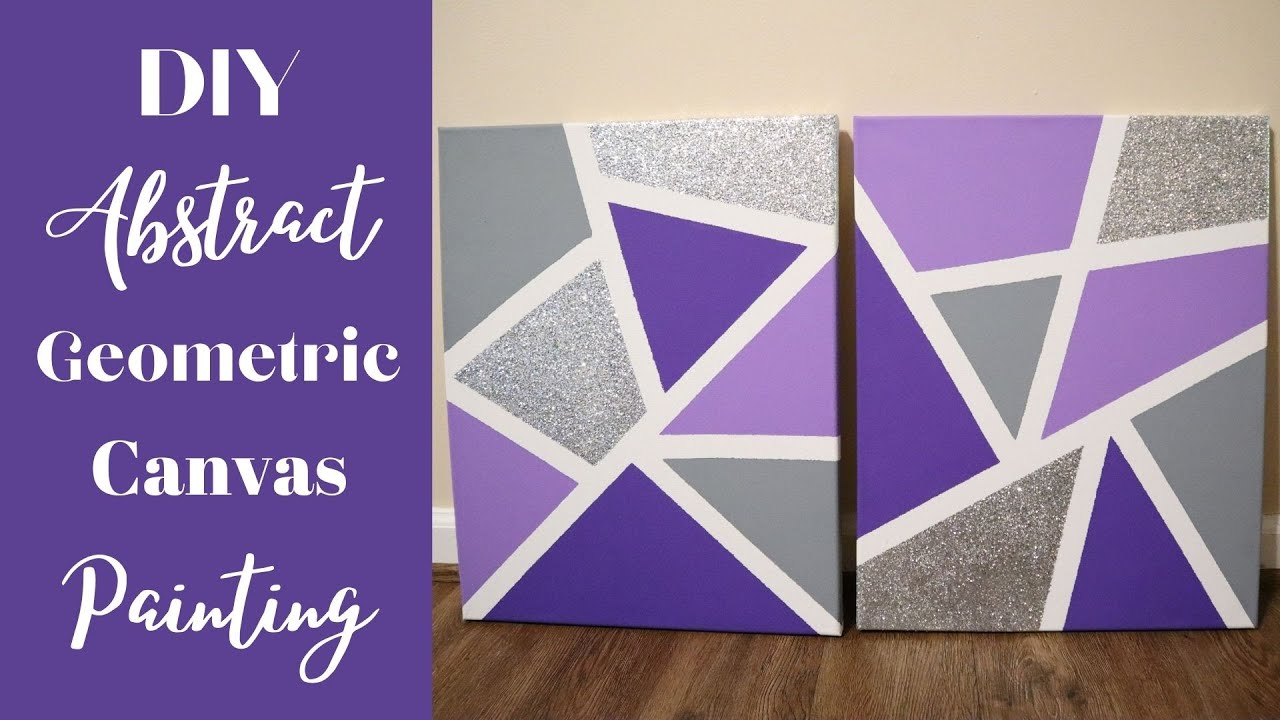The professionally staged indoor photograph, taken under artificial light, features a horizontally rectangular layout with a divided design. The left third of the image shows a solid purple background with white text reading "DIY" at the top in all caps, followed by the cursive word "abstract". Below that, in regular print, are the words "geometric canvas", and the caption concludes with the word "painting" in cursive. The right two-thirds of the image occupy a tan, cream-colored wall with a brown wooden floor. 

In this section, two paintings leaning against the wall are prominently displayed. These canvases showcase abstract geometric designs primarily composed of triangles and various other shapes defined by white lines. The color palette includes shades of light and dark purple, blue, slate gray, and glittery silver. The geometric patterns and the bold, contrasting shapes create a visually dynamic and balanced composition, perfectly exemplifying the DIY abstract geometric canvas painting theme.